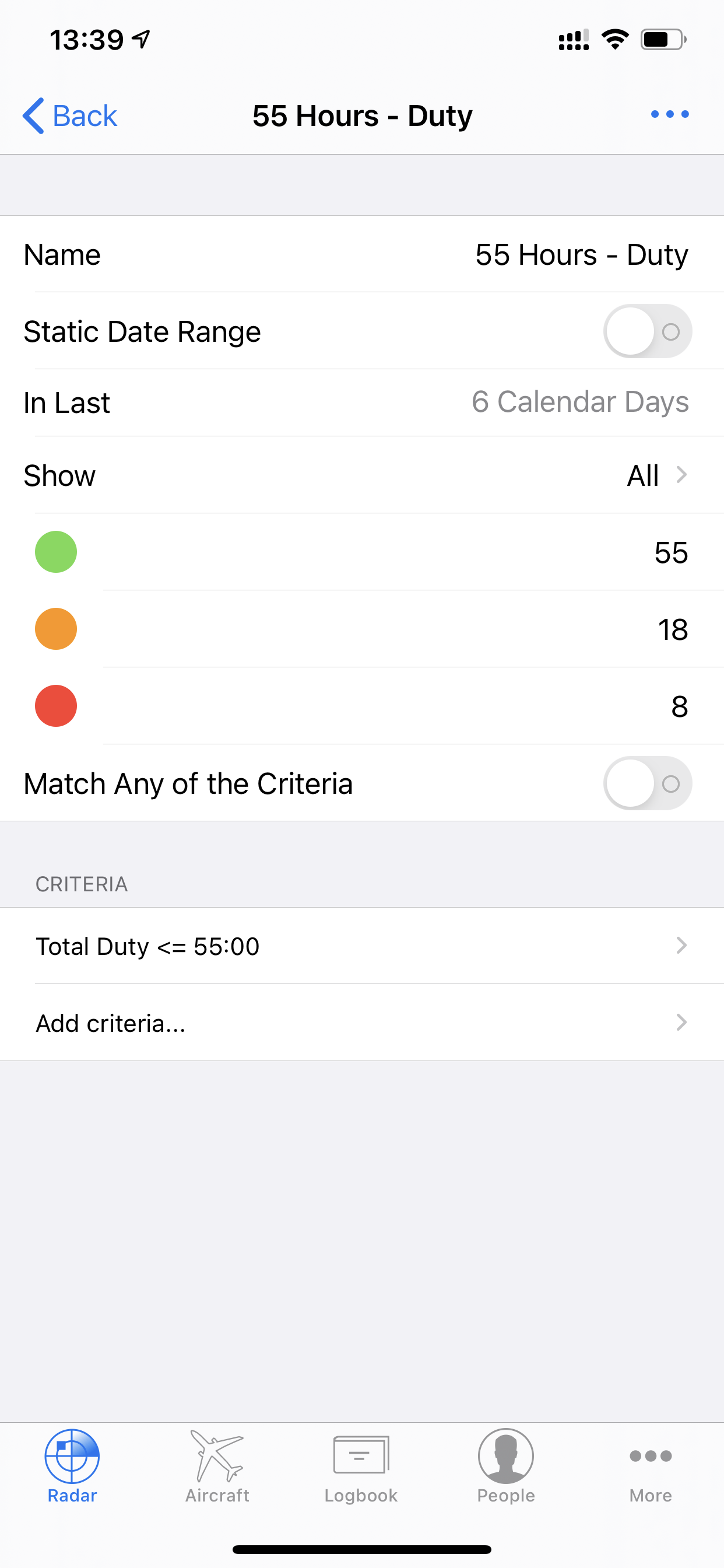This image showcases a detailed view of a cell phone screen interface with a light background. 

**Top Section:**
At the very top left corner, the current time is displayed as "13:39." Adjacent to the time, there's an arrow pointing towards the 2 o'clock position, possibly indicating a notification or a menu. The top right corner of the screen contains several standard cell phone icons, including three or four exclamation marks, a strong cell phone signal icon, and a horizontal battery icon that's approximately three-quarters full.

**Header Section:**
Just beneath the top section, in blue text on the left, there's a left-facing caret accompanied by the word "Back." Centered on this line in dark text, the words "55 Hours Duty" are prominently displayed.

**Main Panel:**
Below this header, there’s a thin, empty gray panel across the screen, dividing the header from the main content area. The information is then presented in a structured format:

1. **First Row of Information:**
   - Left: "Name"
   - Right: "55 Hours Duty"

2. **Second Row of Information:**
   - Left: "Static date range"
   - Right: A toggle button in the off position (white circle moved to the left in a gray oval)

3. **Third Row of Information:**
   - Left: "In last"
   - Right: "Six calendar days" in gray text

4. **Fourth Row of Information:**
   - Left: "Show"
   - Right: "All"

**Key Metrics:**
Below the "Show" category, there are three lines indicating different metrics:
1. First line: Green dot on the left and the number "55" on the right.
2. Second line: Orange dot on the left and the number "18" on the right.
3. Third line: Red dot on the left and the number "8" on the right.

**Additional Settings:**
Following these metrics, there's a line stating "Match any of the criteria" with another toggle button positioned to off (white circle on the left in a gray oval). Below this, a gray line separates the previous section from the next.

**Criteria Section:**
In small gray letters, the word "Criteria" is displayed, followed by:
1. **First White Line:**
   - The text "Total duty is less than or equal to 55:00" in black.
2. **Second Line:**
   - "Add criteria"

Below the "Add criteria" line, there's a large empty gray rectangle.

**Navigation Bar:**
At the very bottom of the screen, there is a navigation bar with five icons and labels from left to right:
1. **Radar** (highlighted in blue)
2. **Aircraft** (in gray)
3. **Log Book** (in gray)
4. **People** (in gray)
5. **More** featuring three horizontal dots above the label, also in gray.

This comprehensive interface likely belongs to a specialized application, possibly used for tracking hours and activities, with various metrics and settings available for the user to customize their view and filters.